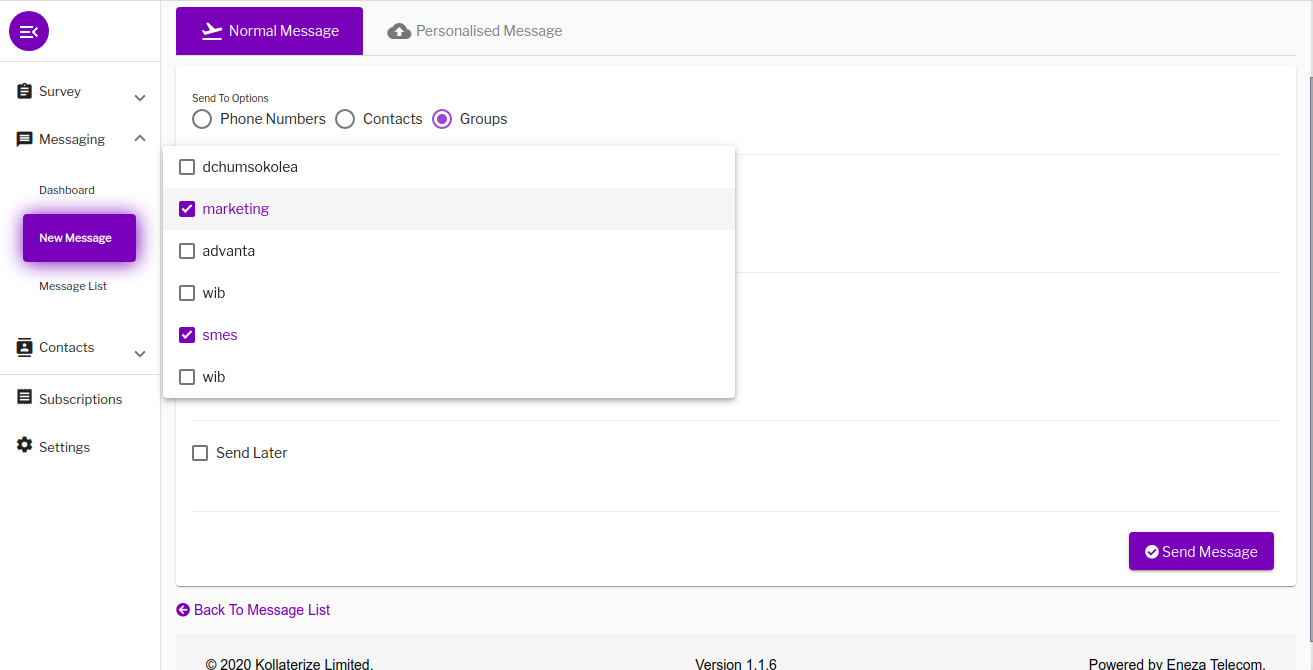**Caption:**

The image displays a user interface, possibly a client management or messaging system, predominantly featuring white, purple, and black colors. On the left sidebar, there is a circular icon with three lines and a downward arrow, indicating a submenu for "Survey," followed by an expanded section labeled "Messages." The sidebar includes menu items such as "Dashboard," "New Messages" (highlighted in purple), "Message List," "Contacts" (with a dropdown arrow), "Subscriptions," and "Settings."

To the right of the sidebar, the main interface shows options for sending messages: "Normal Message" (highlighted in dark purple with white font) and "Personalized Message." Below these options, users can specify the recipients: "Phone numbers," "Contacts," or "Groups," with "Groups" selected, indicated by a purple ticked circle.

Under the recipient options, there is a list with checkboxes for different contact groups. The groups listed include:
- DCHUMSOKOLEA (unchecked)
- Marketing (highlighted in purple and checked)
- Advanta (unchecked)
- WIB (unchecked)
- SMES (highlighted in purple and checked)
- Another WIB entry (unchecked).

The interface appears to facilitate the organization and dispatch of messages, allowing users to select specific groups and customize their communication preferences.